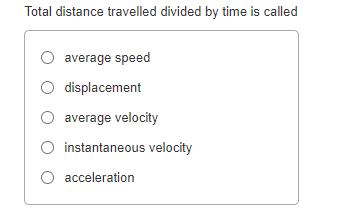The image depicts a minimalistic, grayscale multiple-choice question typically found on a test or questionnaire. The main backdrop is a gray square, which is slightly elongated vertically compared to its width. Within this gray frame, there is a central white box containing the question and possible answers. 

The question at the top of the white box reads: "Total distance traveled divided by the time is called?", and is followed by a list of five possible answers. Each answer is prefixed by an empty circle intended for respondents to fill in their choice. The answers are:

1. Average speed
2. Displacement
3. Average velocity
4. Instantaneous velocity
5. Acceleration

The entire text within the image, including both the question and the answers, is rendered in the same black font. There are no variations in font weight—no bold or italics—ensuring a uniform visual presentation. The stark contrast between the black text and the white background makes the content easy to read despite its simplicity. There are no additional colors, decorative elements, or embellishments, highlighting the straightforwardness and functionality of the image.